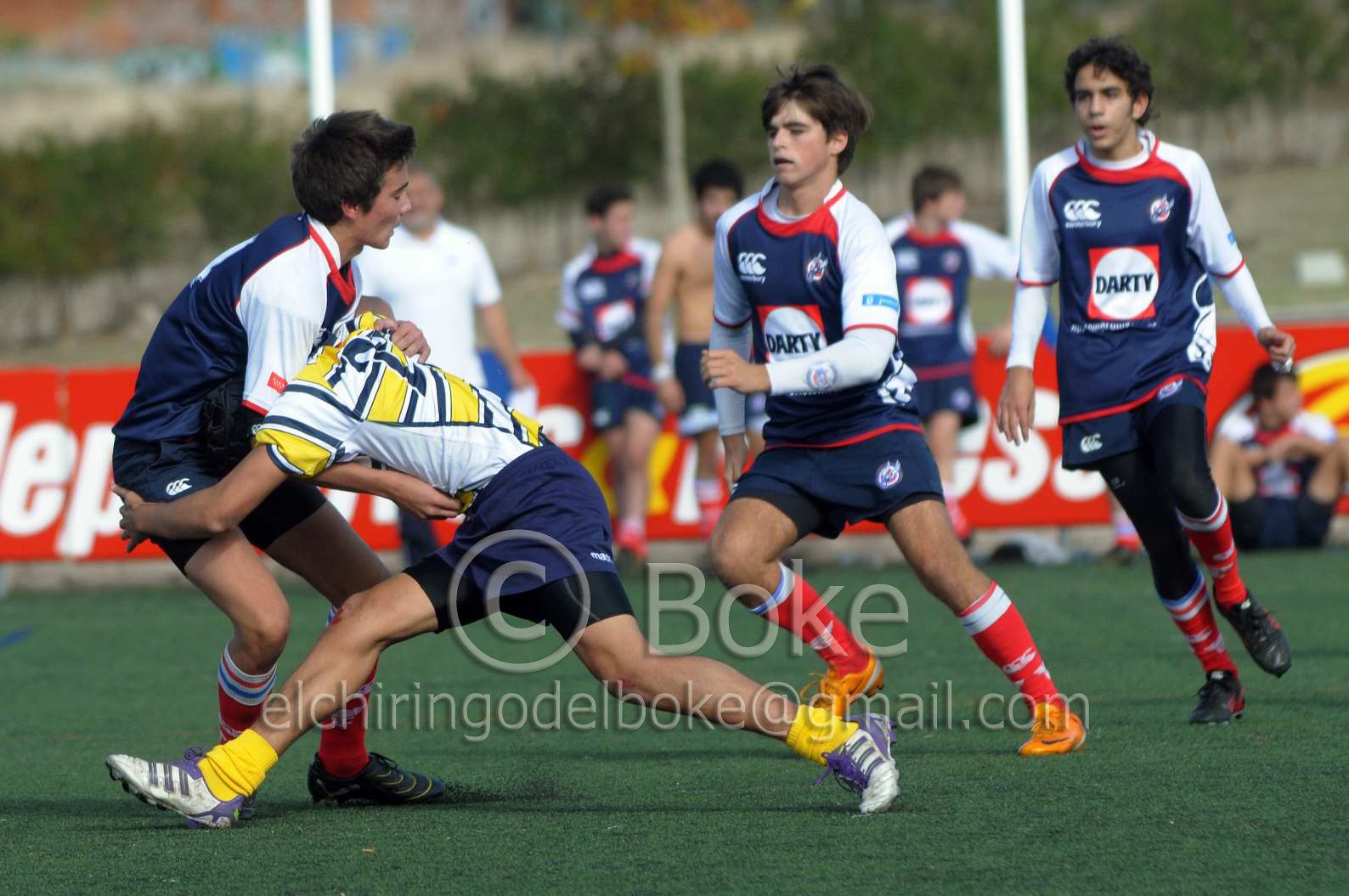This rectangular photograph captures an outdoor rugby match in the midst of active play. Prominently featured in the center of the image are three athletes engaged in a dynamic moment: the player on the left, donning a navy blue jersey with red trim and white sleeves labeled "Darty," is being tackled by an opponent in blue shorts and a distinctive white, yellow, and blue jersey. The player executing the tackle is clad in yellow socks and athletic cleats, typical for the sport. The grassy field forms the backdrop for the action, framed by a divider separating the playing area from the spectator zone, though no stands are visible. Instead, trees and open fields stretch into the distance. Other players, some possibly the team's coach, and one player sitting on the grass, populate the background. The entire scene is overlaid with a semi-transparent copyright symbol and the text "B.O.K.E," along with a partially obscured email address, "Boak Alrick Hiring Godel Boak at gmail.com." The vibrant colors of the uniforms and the green of the grass are prominent, evoking an energetic daytime sports setting.